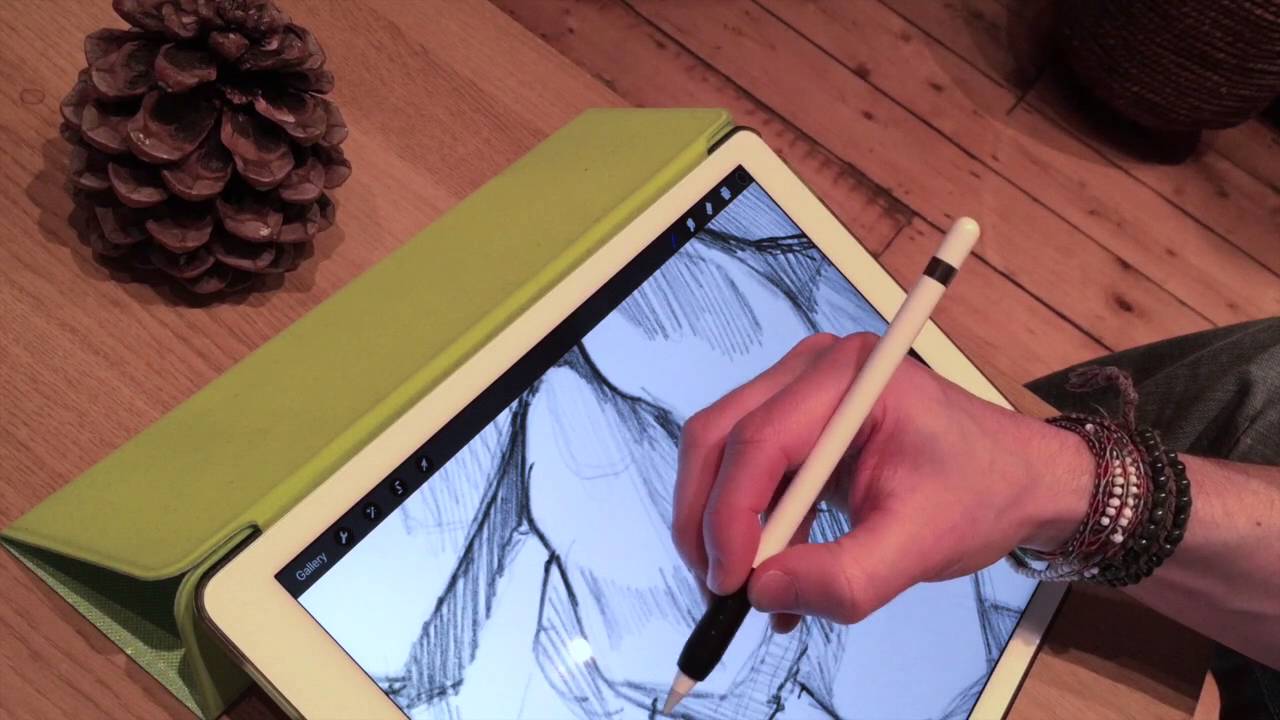In the image, a person with light skin is drawing on a large iPad using a white Apple Pencil with a black tip. The iPad, which has a lime green smart cover folded to act as a stand, is propped up at an angle on a wooden table. The person appears to be sketching a hand, having already shaded some of the fingers, including the fingernails which lack nail polish. The sketch is not entirely clear and may have abstract elements. The artist is wearing several wraparound leather bracelets adorned with black and white beads. Nearby, there are two indistinguishable black items and a pine cone on the table. The scene evokes a homely atmosphere, with the brown wooden table complementing the natural brown of the pine cone.